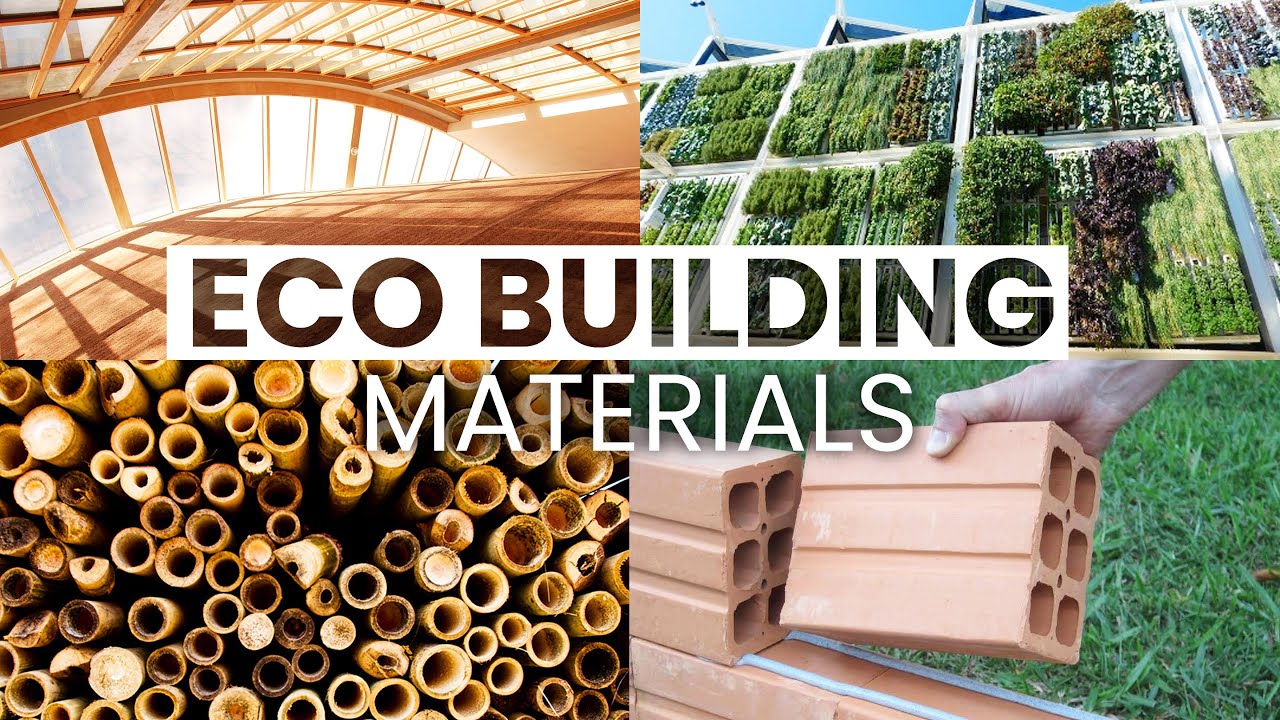The image consists of four photos arranged in a 2x2 grid, serving as a detailed and informative video thumbnail for a topic on eco-friendly building materials. In the top left photo, there is a sepia-toned image showcasing an interior with an arched window framed by wooden materials, suggesting a construction project. The top right photo displays numerous plants growing out from panels affixed to a wall, reminiscent of vertical rooftop gardens or urban agricultural systems. The bottom left photo shows a stack of hollow bamboo rods viewed from their open ends, indicating sustainable construction materials. The bottom right photo features two hands placing together bricks that resemble miniature cinder blocks with six holes. Central to the image is a white rectangle through which the background photos are visible, containing the cutout text "ECO BUILDING" in a brownish sans serif font. Below this, the word "MATERIALS" is written in white letters with a drop shadow, completing the title "ECO BUILDING MATERIALS."